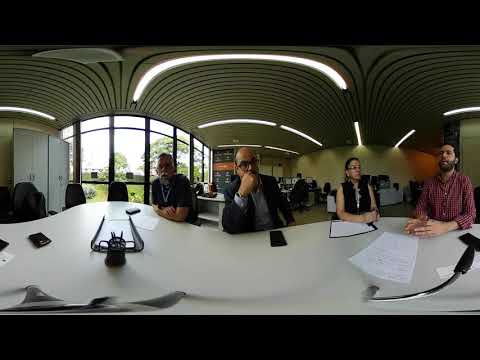This image captures a daytime indoor scene of a group of people seated around a large, white conference table with black wheeled chairs in what appears to be a meeting or hearing. The photograph seems distorted, possibly due to being a still from a panoramic or 360-degree video, resulting in the table and the room appearing curved and warped. Four individuals are seated at the table: an older man with tan skin and a white beard, wearing a black short-sleeved shirt with his arms folded; next to him is a bald man in a black blazer and white button-up shirt, with glasses and one hand covering his mouth; to his right is a woman in a short-sleeved black top and glasses, with papers in front of her; and on the far right, a bearded man with short hair in a red plaid shirt, who appears to be speaking while others listen. The room features broad windows with black grid framing, providing a view of multiple trees and daylight outside. The background includes more desks and tables where another person sits at a computer, two large white cabinets, scattered papers, and wavy-design ceiling lights.